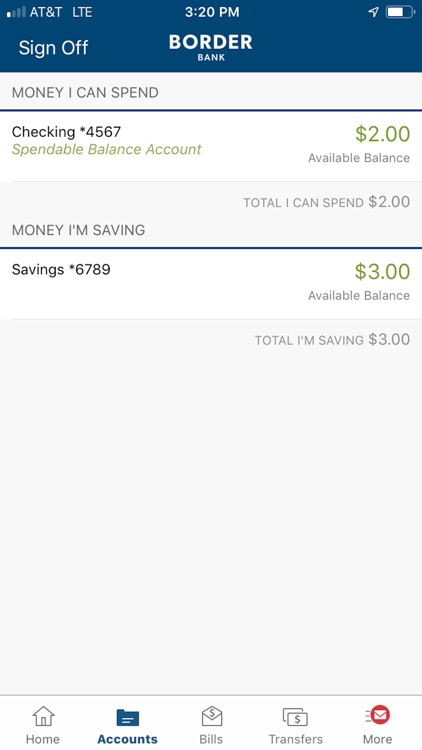This is a detailed digital screenshot taken from a cell phone, displaying the Border Bank mobile app interface at 3:20 PM. The mobile network is AT&T on LTE. The screen shows various financial details starting with "Money I can spend." Within this section, the checking account shows a spendable balance of $2.00 with an account number ending in 4567. The total spendable balance outlined is $2.00. 

The next section is titled "Money I am saving" and features a long blue bar. Underneath, the savings account with an account number ending in 6789, indicated by a small star, shows an available balance of $3.00. The total savings amount is listed as $3.00.

At the bottom of the screen, there is a navigation bar with five buttons: "Home," "Accounts," "Bills" accompanied by an envelope and a dollar sign, "Transfers" shown with a dollar sign over money, and a "More" button, stylized in red and white with an envelope icon.